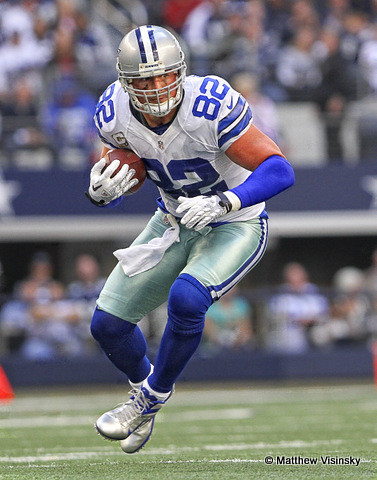The photograph captures an NFL football player mid-action, seemingly floating in the air with both knees bent as he runs. The player is most likely Jason Witten from the Dallas Cowboys, recognizable by his blue and white team colors. He is wearing silver-colored football cleats with white laces, blue leggings, and silver shorts with white and blue stripes on the sides. His outfit includes a white jersey with prominent blue stripes on the sleeves and a blue number 82 displayed on the front and shoulders. A blue belt with a white towel hanging from it accentuates his uniform. The photograph marvelously freezes the moment as he holds the football in his right arm, ready to juke away from a tackle while extending his left arm to fend off opponents. The green, closely-cut grass beneath him contrasts with the blurred audience in the background, highlighting his intense action. Completing his ensemble is a helmet and full NFL gear, epitomizing a quintessential football play. The bottom right corner of the image discreetly bears a copyright notice in black text reading "copyright Matthew Vysinski."